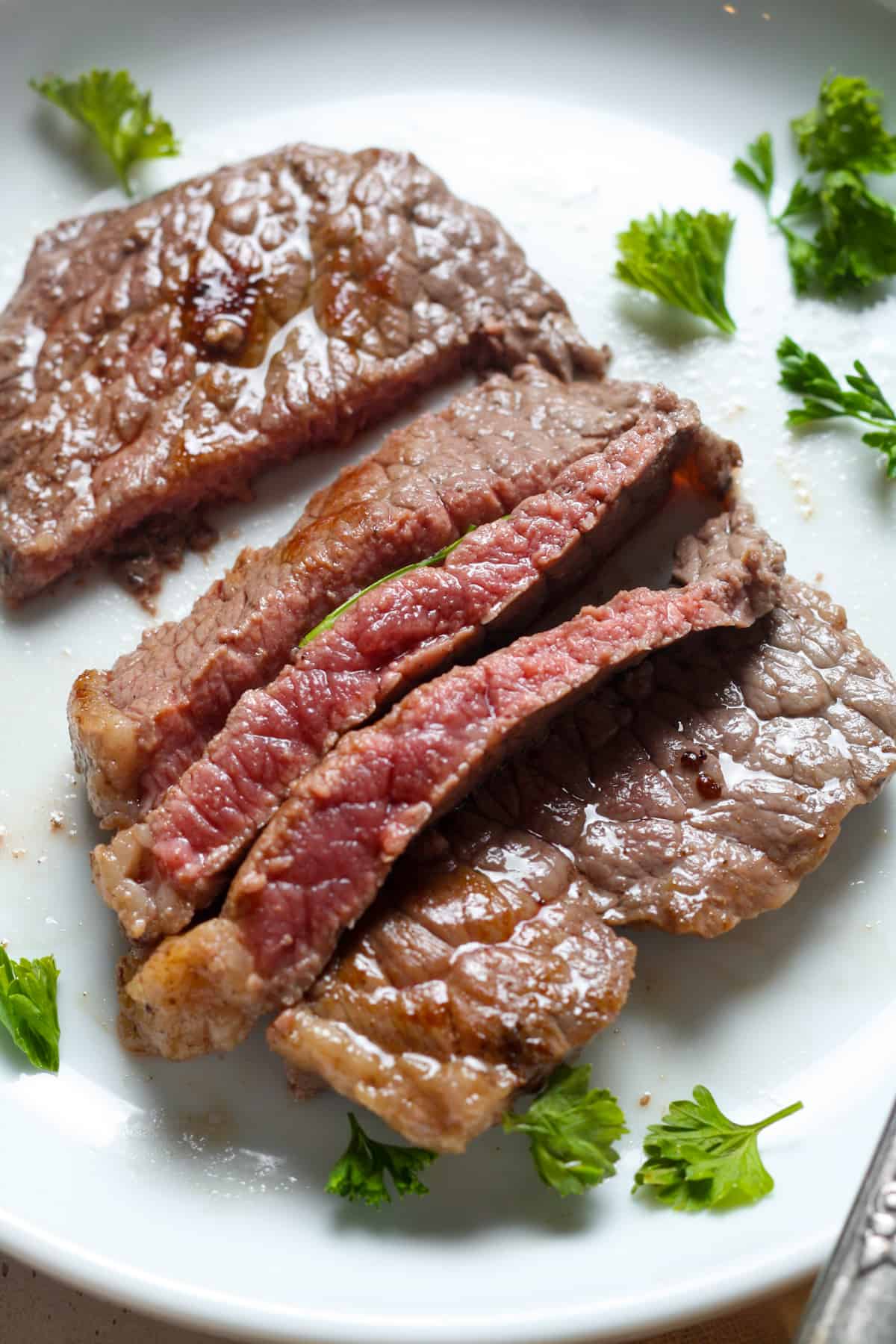This detailed close-up photograph showcases a small, medium-rare steak, positioned centrally on a pristine white plate. The meat is distinctly cut into multiple segments: the ends remain whole while the center is sliced into three or four thin strips. Each piece exudes a succulent, juicy appearance with visible reflections of moisture, enhanced by the natural pink hues and slight charring on the surface. The steak is garnished with delicate green celery leaves and parsley snippets that add a fresh, vibrant contrast to the dark red and brown tones of the meat. In the bottom right corner, a silver utensil subtly peeks into the frame, emphasizing the dish's ready-to-eat appeal. Overall, the photograph, likely taken by a photographer with a focus on food presentation, presents the luscious steak in an overhead view, making the succulent texture and rich colors the centerpiece of this elegant culinary capture.